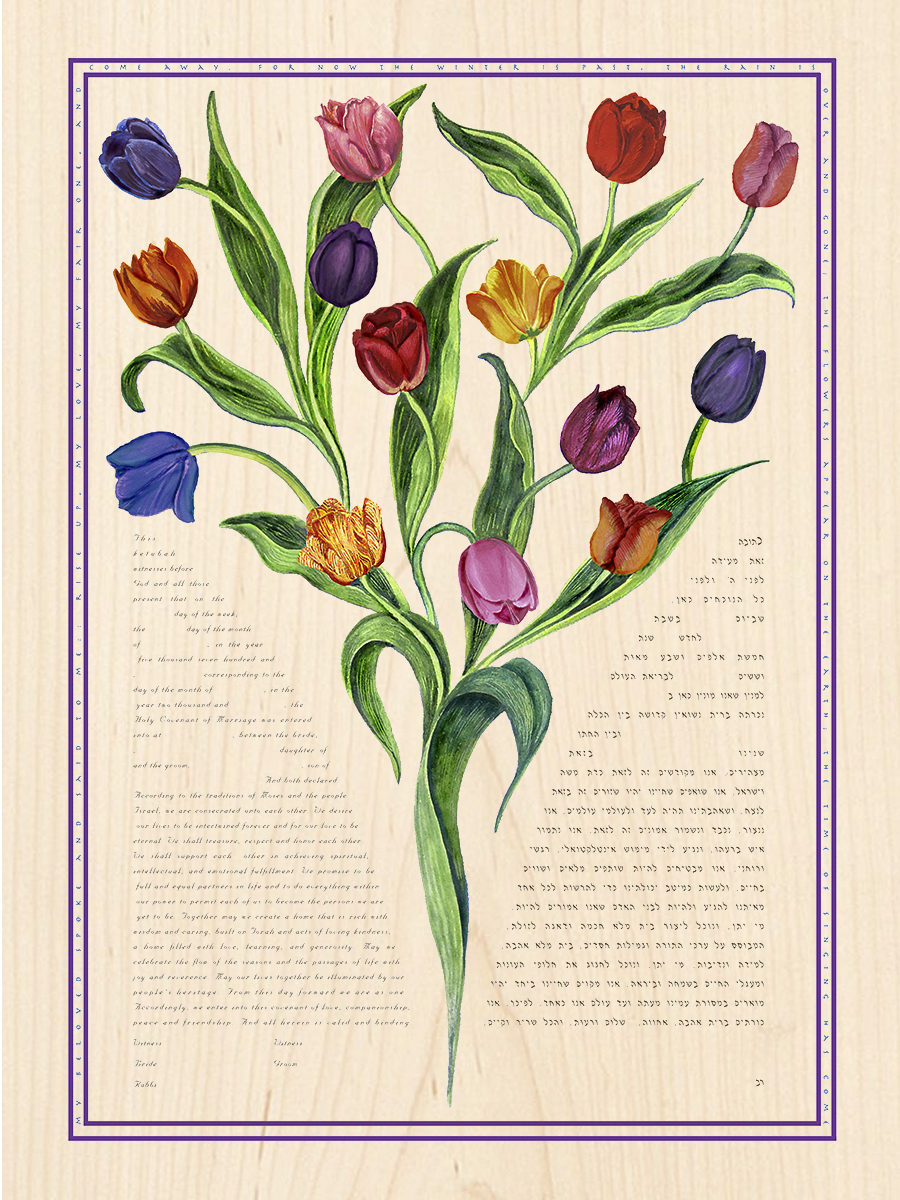This detailed illustration features a vibrant bouquet of flowers set against a pale beige, wood-toned background. The image is framed by two closely spaced, purple rectangular borders decorated with light blue dots in between. The central focus is an array of flowers and foliage, with pink, orange, yellow, red, blue, and various shades of purple blooms, including roses and tulips, all emerging from green stems and leaves that ascend from the bottom to the top of the image. These flowers are depicted in multiple stages of bloom, with some petals curling and others standing tall. 

Text in an artistic curve, too small to read clearly, encases the flowers, written in English on the left side and appearing to be in Hebrew on the right, forming a mirrored, yet symmetric pattern. The text, partially readable, includes phrasings like "come away for now the winter is past the rain is..." and continues with other lines. The artistic rendering is found on either page 21 of a book or a magazine, emphasizing both artistic and literary elements in its presentation.